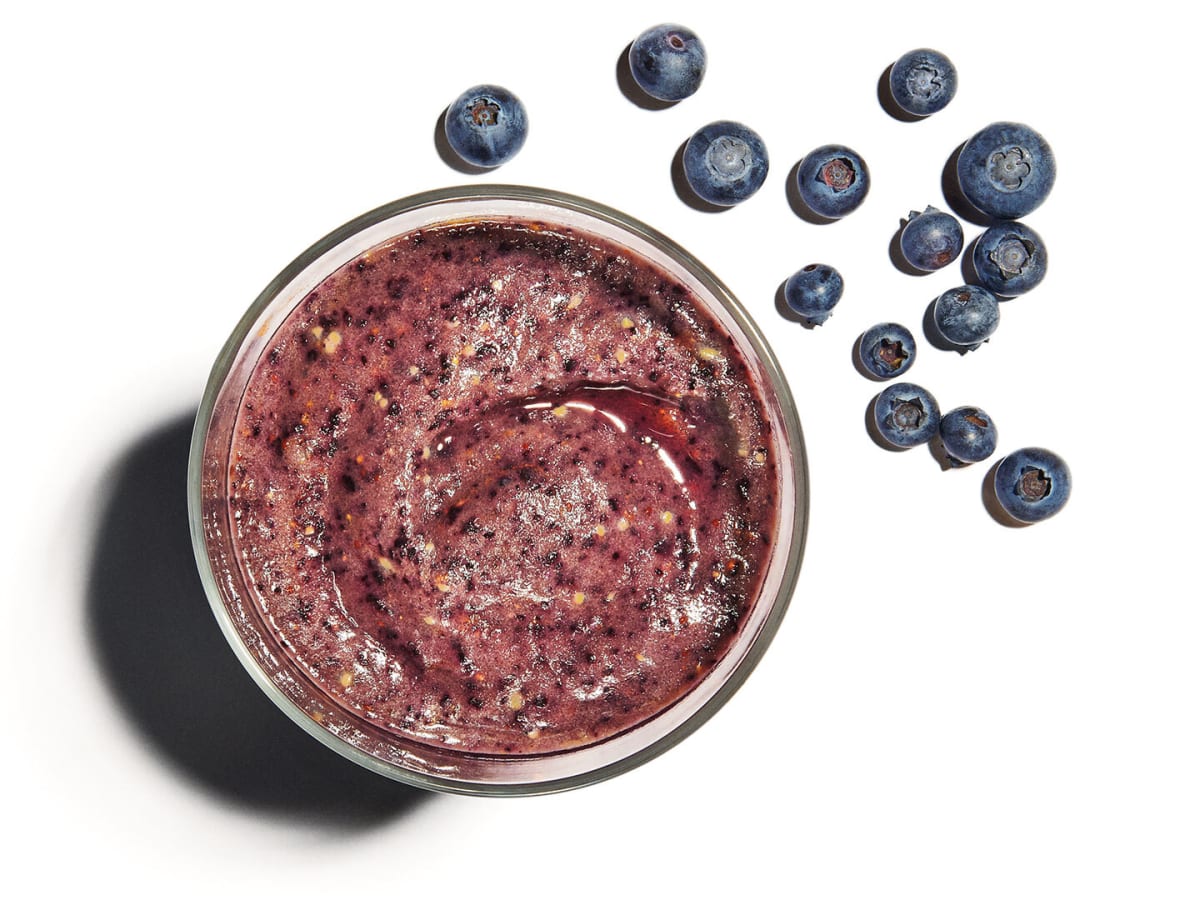In this simple, color photograph set against a completely white background, we see an artful arrangement of blueberries and a blueberry-based dessert from a top-down perspective. Scattered from the top center to the right and down to the right center are fourteen blueberries of various sizes, some even showing the brownish remnants of their stems. Dominating the left side of the image is a small, clear glass bowl containing a richly colored blueberry custard or dessert. The dessert is a mixture of blue and purple hues, with noticeable specks of darker blue, which are likely blueberry skins, and flecks of white. A slight accumulation of purple liquid is swirled to one side of the bowl, enhancing the appetizing, possibly healthy nature of the treat. The detailed display suggests it could easily be a professional food photograph for a recipe or advertisement promoting blueberries.